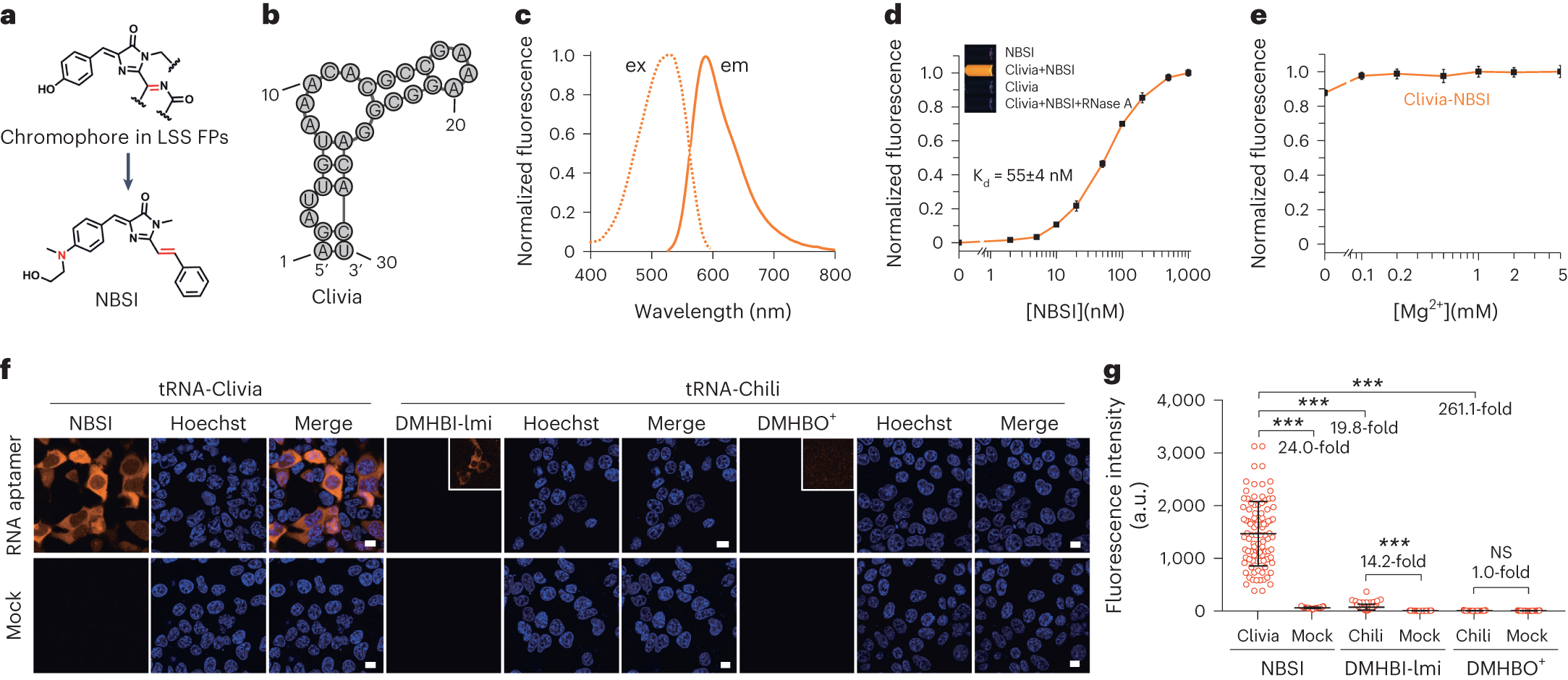This image appears to be a detailed scientific figure from an educational resource such as a textbook or science test, focusing primarily on tRNA and various fluorescence measurements. It comprises multiple labeled sections (A through G) on a white background, containing a mix of graphs and microscopic images. 

Sections A and B include diagrams and hexagonal figures with terms such as "chromophore" and "colivia," alongside structural representations. Section C features a graph measuring normalized fluorescence against wavelength, while sections D and E contain scatter plots quantifying normalized fluorescence relative to NBSI and Mg²² respectively. 

Section F offers a visual comparison of RNA samples, including mock and tRNA colivia, depicted in purple, pink, and black colors through microscopic imagery. Finally, section G presents another scatter plot, assessing fluorescence intensity across various substances (DMHBI, DMHBO, and NBSI). The graphs are characterized by black text with prominent orange lines and accents, creating a comprehensive visual aid for understanding the scientific data presented.